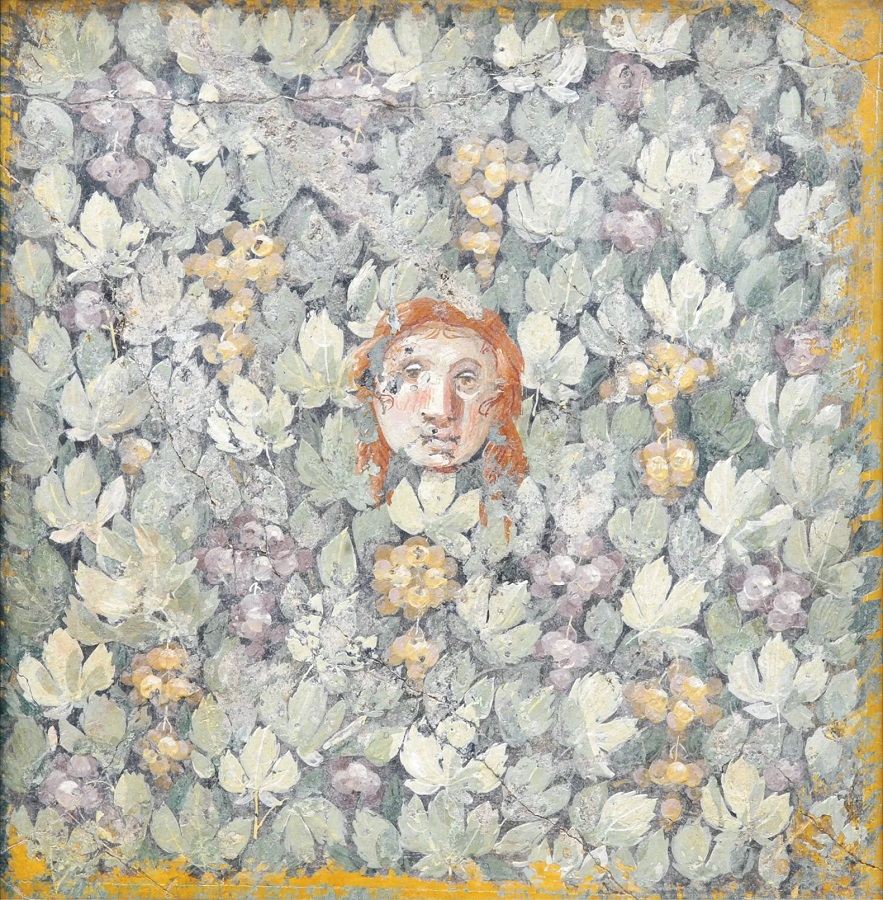The image features a captivating painting of a young girl’s face, prominently positioned in the center of the artwork, which is slightly rectangular, about six inches high and five inches wide. The girl has a distinctly round face with very light, almost pasty skin that shows faint red undertones from underlying blood vessels. Her facial features are well-defined: she has a broad nose, small, spaced-out, round-shaped eyes shaded with heavy eyelids, brown irises, a closed mouth with thick lips, and a small chubby chin. Her reddish hair frames her face, appearing to flow down the sides, somewhat resembling pigtails.

The girl's head appears to be emerging from a vibrant bed of flowers and leaves, a surrealistic juxtaposition that adds depth and intrigue. Surrounding her face are predominantly orange and purple flowers, with pale green leaves that have a five-section structure similar to maple leaves. Scattering these leaves and flowers are small yellow balls or grape-like clusters of light purple and golden hues, creating a sense of richness and density. The outer edges of the image are accentuated with paint strokes in mustard-yellow tones, suggesting a border that frames the entire composition. The texture seems almost cracked, giving the impression that the painting might be on a stone canvas. Together, these elements create a mesmerizing and intricate visual experience.